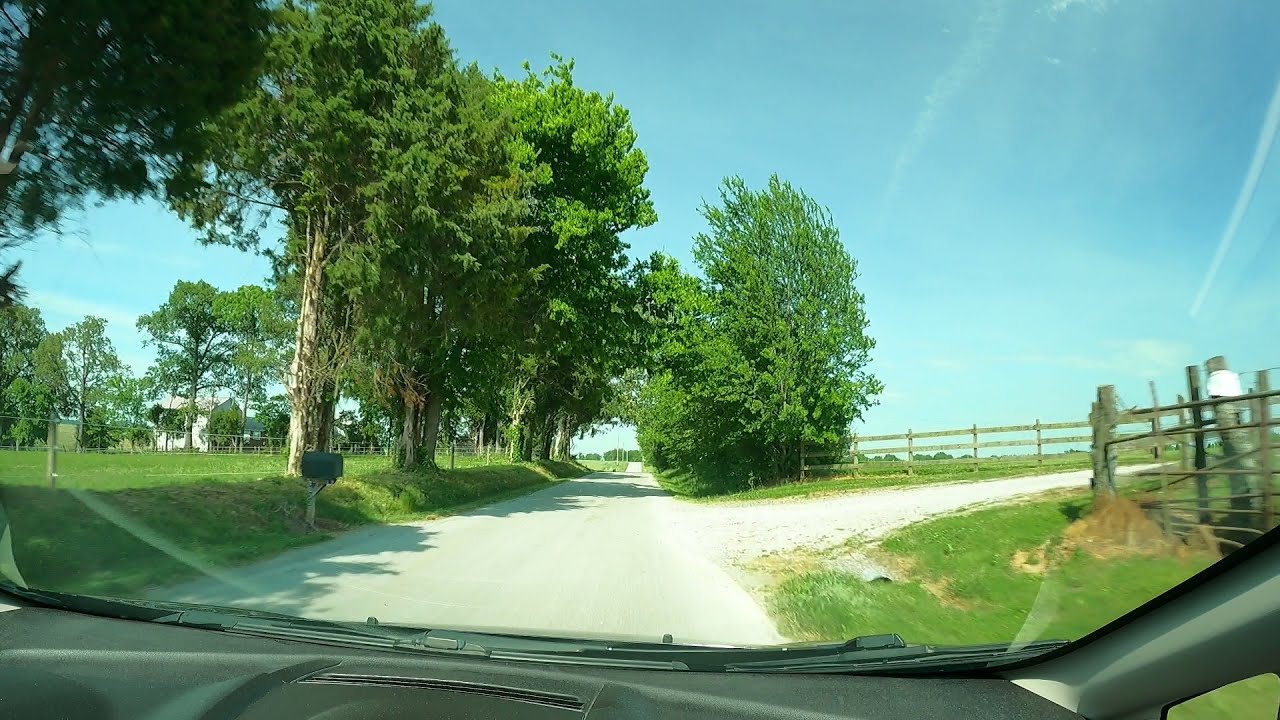This horizontally aligned rectangular photograph, taken from inside a vehicle with visible glares on the lower left and upper right parts of the windshield, showcases a serene country road scene. The car's dashboard is a darker gray color, and the windshield wipers are visible. The road, appearing either paved or smooth, stretches ahead, flanked by tall green trees on both sides. To the right, there is a gravel road that seems to lead to a farm area, marked by wooden rail-type fencing. Near this turnoff, a black mailbox stands out conspicuously. Both sides of the road feature grassy areas with trees, and there's another wooden fence on the left, along with an expansive lawn. In the distant background, a white house is faintly visible. The sky is a clear blue, accented by a few feathery clouds and contrails from aircraft, contributing to the tranquil rural atmosphere.